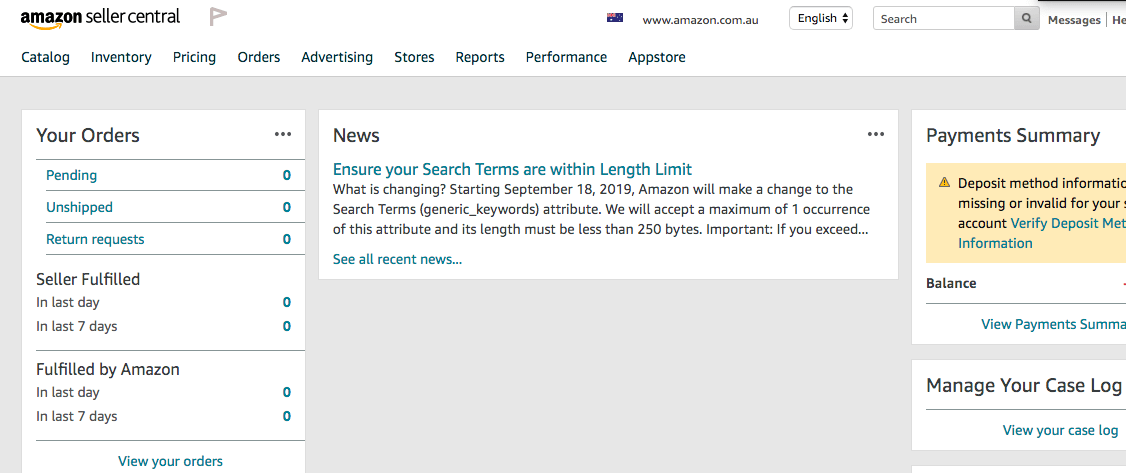The image displays a screenshot of the Amazon Seller Central page with a clean white background. In the top left corner, the Amazon logo is prominently placed, followed by the "Seller Central" label. To the right, a grey flag icon can be observed in black text, indicating a language or regional setting.

On the top right corner of the page, there is an Australian flag icon accompanied by a URL link directing to Amazon Australia. Adjacent to this, a language selector box set to English is visible, featuring up and down arrows for navigation. Immediately next to the language selector, there's a search box with grey placeholder text and a grey magnifying glass icon indicating its purpose. Further right, the word "Messages" appears in grey text, separated by a grey vertical line from a partially visible word beginning with the letter 'H'.

Below this, there is a navigation menu in blue text listing the categories: Catalog, Inventory, Pricing, Orders, Advertising, Stores, Reports, Performance, and App Store, arranged in a single row.

Directly beneath the menu, a sizable grey box is divided into three columns: "Your Orders" on the left, "News" in the center, and "Payments Summary" on the right. Each of these sections includes a three-dot menu icon in the top right corner for additional options. Within these boxes, both blue and grey or black text are used to convey various pieces of information related to each category.

Additionally, near the bottom of the page, there is another separate box titled "Manage Your Case Log," suggesting options to handle open support cases or issues.